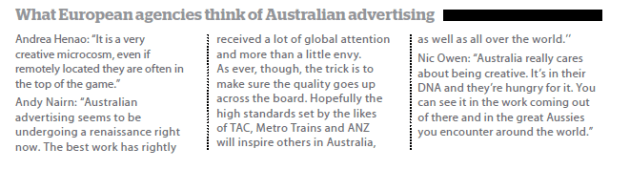**What European Agencies Think of Australian Advertising**

The image features black text on a white background with three columns of text separated by thin dotted lines. The content is concise yet quite small, requiring enlargement for easier reading. 

At the top of the page, there's a headline: *"What European Agencies Think of Australian Advertising."* Directly beside it, a few words are obscured by black redaction marks. 

Within the columns:

- **Left Column**: The text begins with *"Andre Haino"* offering commentary enclosed in quotation marks: *"It's a very creative microcosm. Even if remotely located, they're often at the top of the game."*

- **Middle Column**: The commentary continues with *"Andy Nairn"* stating: *"Australian advertising seems to be undergoing a renaissance right now. The best work has rightly received lots of global attention and even more than a little envy. As ever though, the trick is to make sure the quality goes up across the board. Hopefully, the high standards set by the likes of TAC, Metro Trains, and ANZ will inspire others in Australia."*

- **Right Column**: Lastly, *"Nick Owen"* shares his thoughts: *"Australia really cares about being creative. It is in their DNA and they're hungry for it. You can see it in the work coming out of there and in the great Aussies you encounter around the world."*

The overall layout resembles an excerpt from a newspaper or magazine, with the structured columns and thin dotted lines enhancing readability.